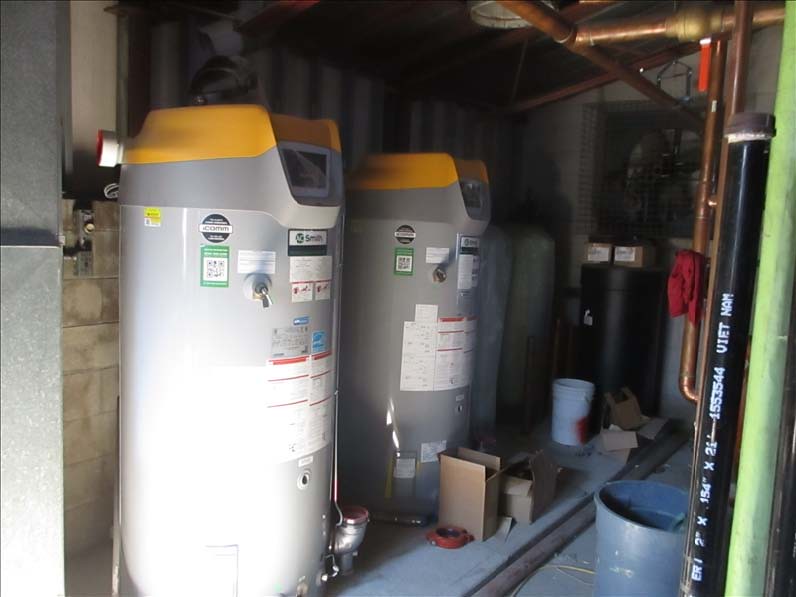This is a detailed photograph taken in a partially finished utility room, with light filtering in through an open door. The room's walls are unfinished, with the lower parts made of concrete blocks, and the floor also concrete. Visible in the image are multiple pipes, including black and brass ones, and copper-colored pipes running along the ceiling. Dominating the middle left are two identical cylindrical structures, likely water heaters or softeners, with gray bodies and yellow tops, adorned with various unreadable stickers. A large green pole stands beside a black pole labeled "ER2X154X2" and "Vietnam" in white writing. Towards the back, a significant industrial fan is visible. The ceiling features brownish pipes, enhancing the unfinished look. Miscellaneous items scattered on the floor include cardboard boxes, a white bucket with red spray paint, and a red clamp.